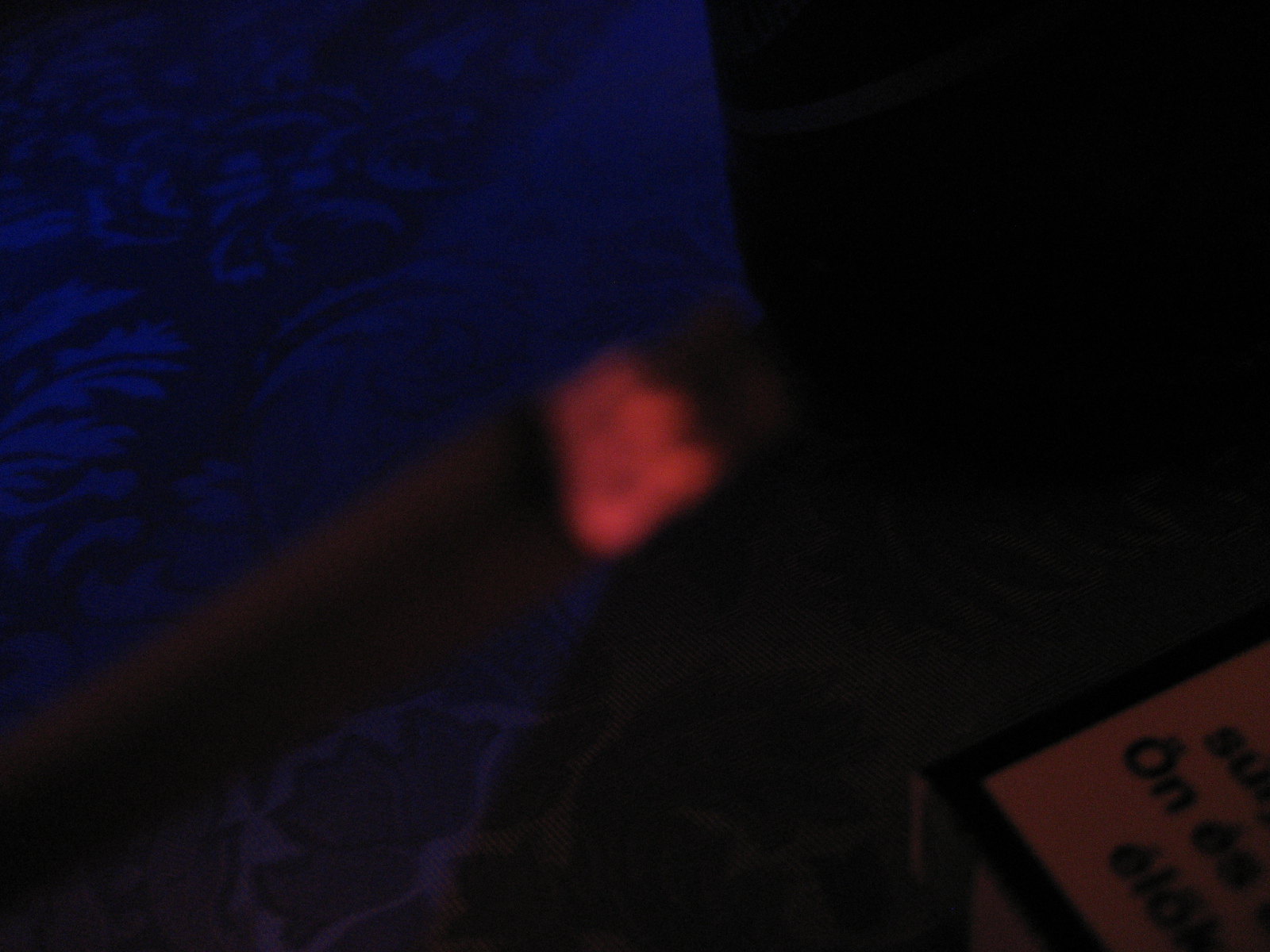This photo depicts a very blurry, dark scene primarily featuring the lit cherry of a cigarette with an embery red glow and some ash at its end. The background is difficult to discern but shows some details that barely emerge through the haze. The upper left corner appears to show plants and possibly a window with a flowery, black-and-blue design, hinting at either an indoor setting or a view looking outwards. A faint blue hue can be seen in this area. The center of the image features a red light, contributing to the overall darkness. To the right, there is a sign with partially legible lettering, "O-N," against a white backdrop. The scene might be set at night, further shrouded in indistinct shadows and hues of black, blue, and red.